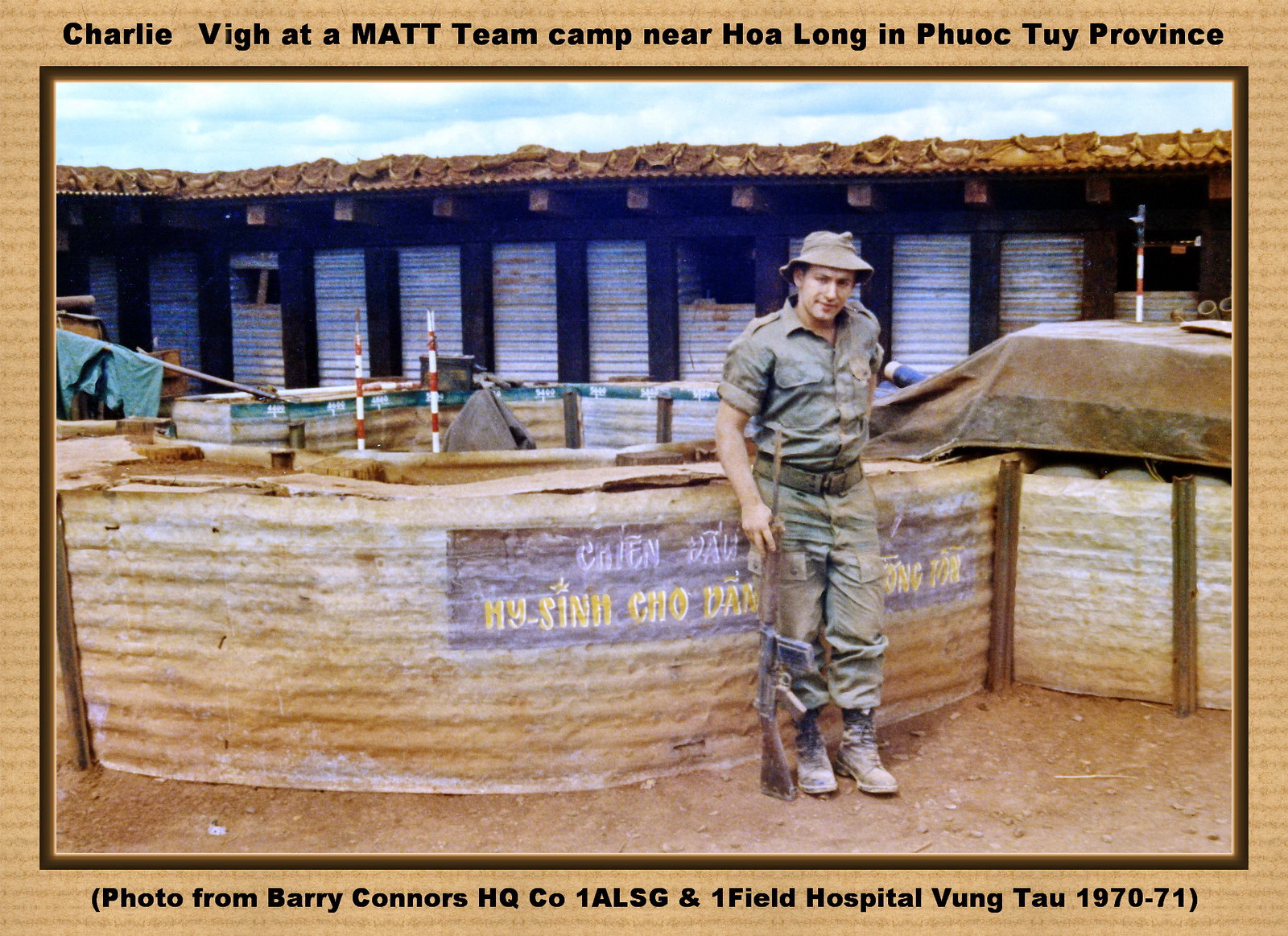This outdoor photograph captures a man standing on the center left, dressed in green military garb complete with a belt and a hat. In his right hand, he holds an assault rifle, which rests on the ground beside him. The backdrop features a makeshift barrier and several storage sheds, hinting at a military camp setting. Above the photograph is a caption that reads, "Charlie Vinn at a MATT team camp near Howe Long in Phuoc Tuai province," while the bottom caption states, "Photo from Barry Connors HQ, Co. 1ALSG in Onefield Hospital, Vang Thao, 1970-71." Furthermore, a partially visible sign behind the man reads "MICE and CHO." The sky appears overcast, adding a muted tone to this historical military scene.